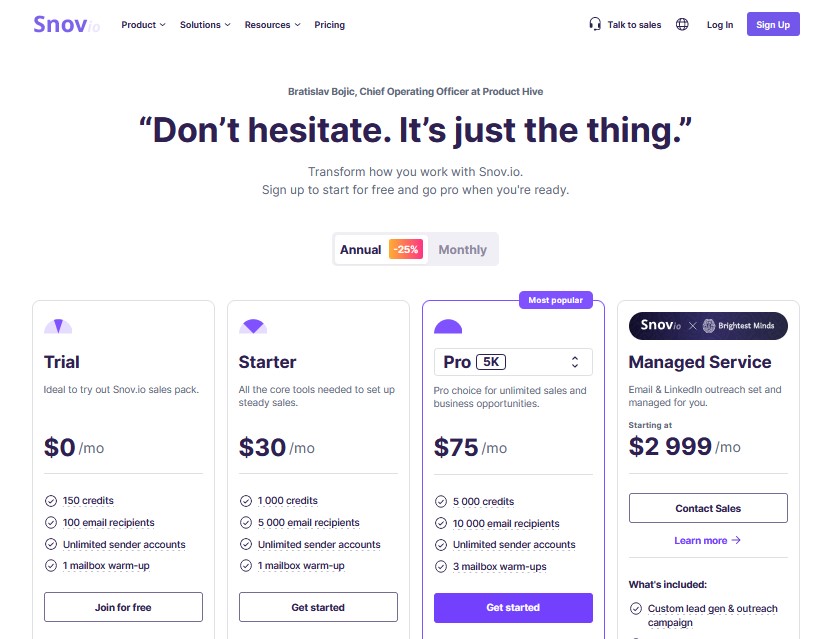The image captures promotional content for SNARV, showcasing their offerings for podcast solutions, resources, and pricing structures. Here’s the refined and detailed caption:

---

"Promotional material for SNARV detailing its podcast solutions, resources, and pricing plans. The content prominently features:

1. **Practice & Resources:** Mentioning a Chief Operating Officer at Productive Hive, suggesting high-level expertise.

2. **Call to Action:** Encourages users to 'Transform how you look and work with snarv.io.' It prompts users to sign up for free to start and to upgrade to a pro plan when ready.

3. **Pricing Plans:**

   - **Trial:** Free, ideal for trying out SNARV.IO's sales pack.
   
   - **Starter Plan:** Priced at $30 per month, includes all core tools needed for establishing steady sales.
   
   - **Pro 5K Plan:** Costs $75 per month, suitable for those seeking ultimate sales and business opportunities.
   
   - **Managed Service:** At $2,999 per month, SNARV offers premium managed services, including email and LinkedIn outreach managed by 'SNARV’s brightest minds.'

The information emphasizes a strategic hierarchy of services designed to cater to varying business needs, from initial trials to comprehensive managed services."

---

This caption provides a structured and thorough overview of the content in the image, making it accessible and informative for the reader.